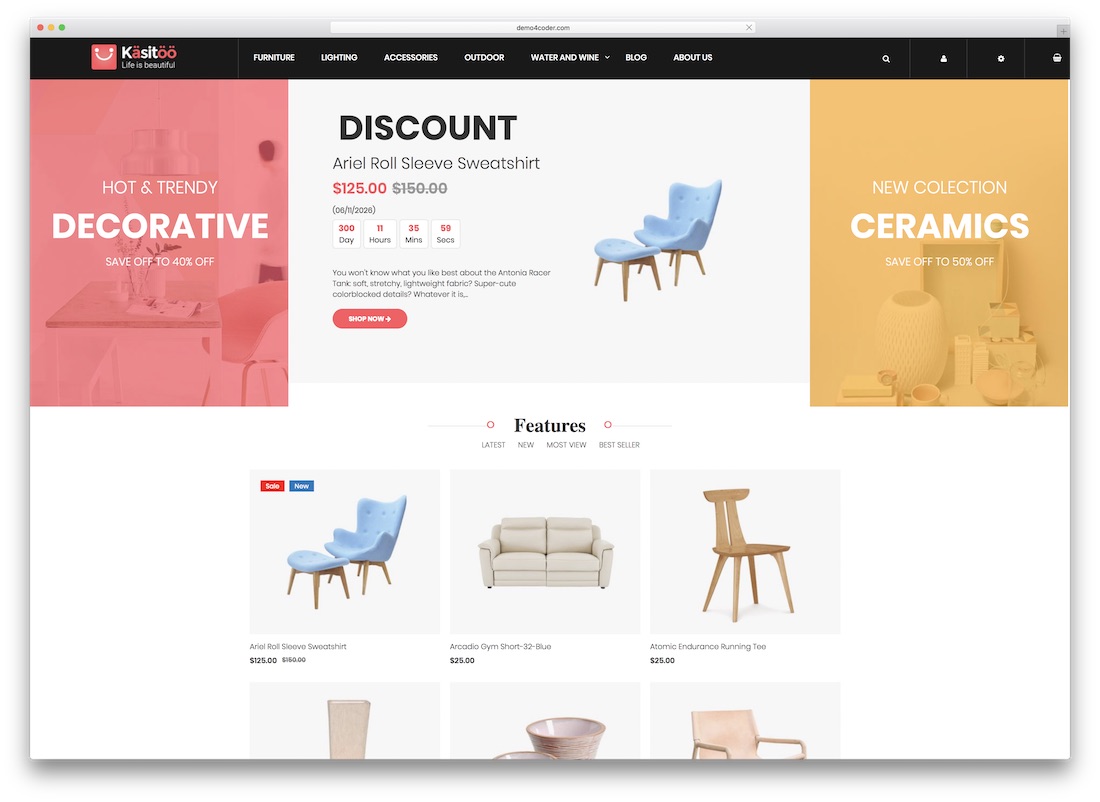The image features a complex, visually rich layout with a variety of geometric shapes and UI elements. Here's the detailed description of the image:

---

At the top of the image, there is a prominent gray rectangle spanning the width of the layout. On the left side of this rectangle, there are three circular icons: a salmon-colored circle, a yellow-orange circle, and a green circle. Centrally positioned within this top area is a white rectangle containing text and an ‘X’ icon on its right-hand side, suggesting a close button or dismiss option.

Below this gray rectangle is a small gray square or rectangle with some indistinct content. Directly underneath, there is a black rectangle. Adjacent to these elements on the left side is a salmon-colored square displaying a smiley face icon, accompanied by text in a mix of white and salmon color.

Proceeding downward, there are white words that are somewhat illegible. Further along, the layout features an icon likely representing a magnifying glass, followed by two ambiguous symbols, and finally an icon resembling a lock.

Positioned on the left beneath these icons, there is a salmon-colored rectangle with an image that appears to showcase furniture. The text within this rectangle reads “Hot and Trendy, Decorative, Save Up to 40%”. To its right is a gray rectangle with the wording “Discount, Aerial Roll, Sleeves, Sweatshirt, $125.00,” beside which is the crossed-out price "$150.00". 

Further down the layout, there are four white squares. Each square contains a red element at the top that may be a number or word and a black text at the bottom. Additional words in black or gray text are present but unclear from the description.

Continuing downward, there is a salmon-colored rectangle with slightly bulging sides. It contains text and features an image of a blue chair with a matching blue stool. Adjacent to this is a dark yellow rectangle with an indistinct image labeled “New Collection, Ceramics, Save Up to 50% Off”. Below this, the word “Features” appears in the center, flanked by two red outlined circles—one on the left and one on the right. 

Below the "Features" section, the blue chair reappears within a salmon-colored rectangle and a blue rectangle with accompanying text. To the right, there is an image of a sofa, followed by another picture of a chair. At the bottom left, partly visible, there is an image too cropped to identify, likely ceramics. The sequence ends with another partial image suggesting a chair.

---

The description captures the intricate design and varied content, organizing it in a structured manner for clearer understanding.